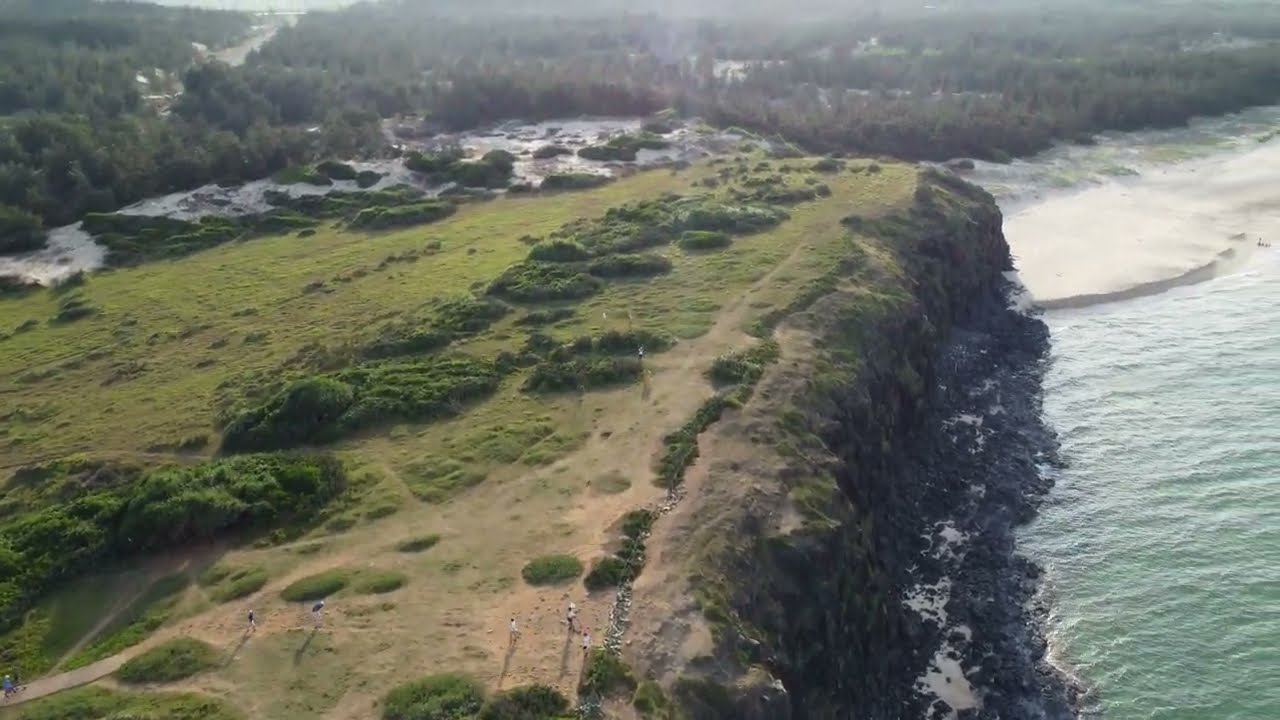This vibrant aerial photograph, captured by a drone approximately 200 feet above, showcases a dramatic seaside landscape in breathtaking detail. The centerpiece is a massive rocky cliff that plunges directly into the ocean below, with jagged black rocks scattered along its base, likely fallen from above. The ocean displays a deep greenish-blue hue, with white foam visible where the waves crash against the cliffside. 

The cliff, estimated to be around 60 feet tall, is covered with patches of green grass, low shrubs, and naturally forming dirt paths from frequent foot traffic. On top of the cliff, about ten people can be seen, engaging with the landscape. To the top right of the image lies a serene sandy beach with pristine white sand and no visible visitors, backed by a small neighborhood nestled within a forest area. In the far top left corner, a two-lane road can be seen indicating access to this remote yet scenic location. The lush vegetation in the distance adds to the view's richness, offering a glimpse of thick forests that stretch across the top edge of the image.